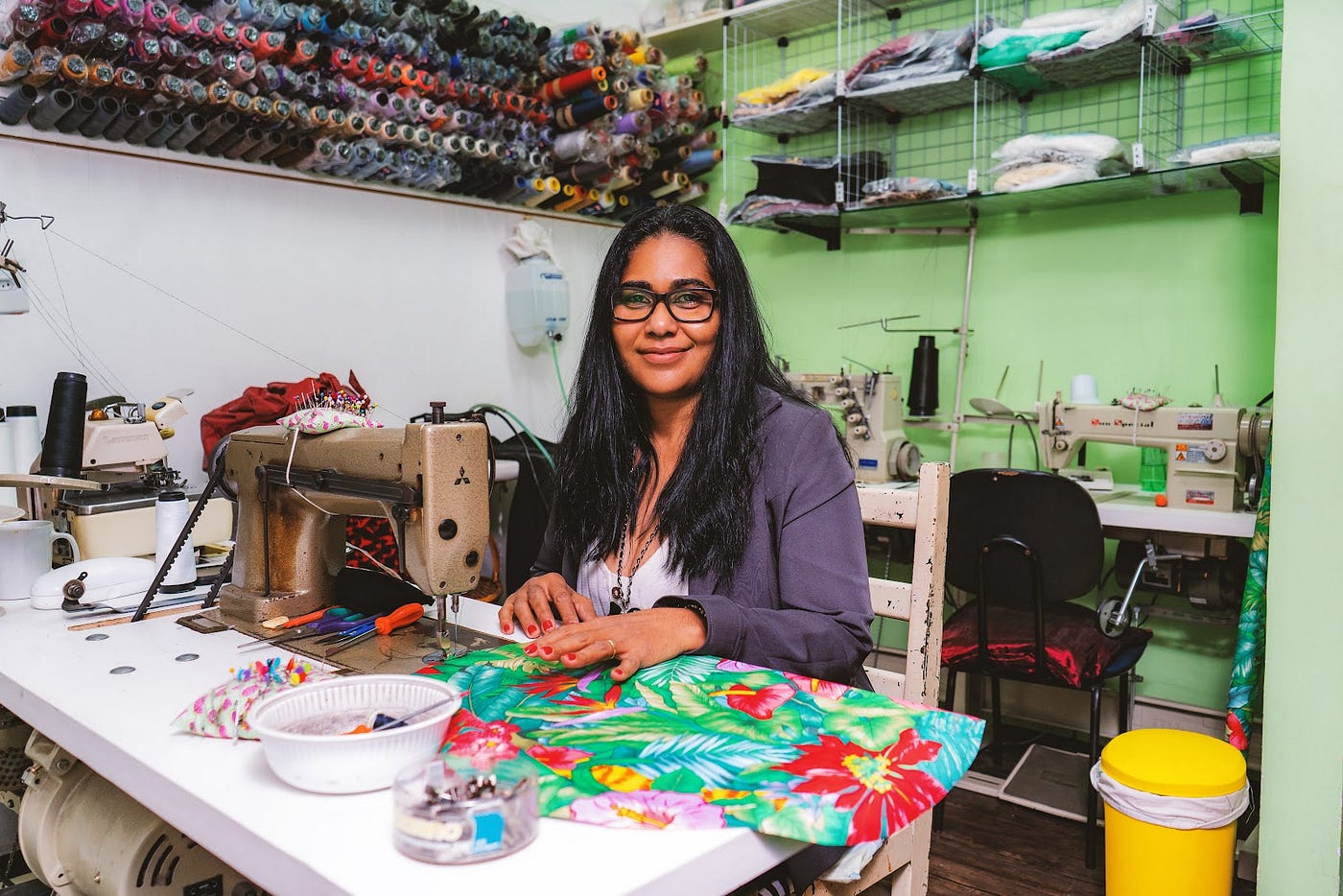This photograph captures an African or African American woman, likely in her 30s, seated at a sewing station, smiling and looking directly at the camera. She has dark brown skin, long black hair that cascades past her chest, and wears black-framed glasses. Her attire includes a white shirt underneath a bluish-purple jacket, accessorized with several necklaces.

She is seated on a white chair at a white table, which holds an old, bronze-colored sewing machine. In front of her is a vibrant Hawaiian-patterned fabric featuring red flowers, green leaves, and possibly yellow and orange fish, draped across the machine as she works. The table is cluttered with various tools essential to her sewing craft, including an orange-handled screwdriver and metallic objects.

Surrounding her workspace, the wall on her left is white and adorned with an array of colorful thread spools neatly stacked. To her right, a green wall features shelves filled with folded materials and various items wrapped in plastic. Behind her is another white desk with a white sewing machine and a black chair. A distinctive yellow wastebasket lined with a white bag sits on the floor to her right. This professional-looking sewing area suggests a bustling and organized environment.